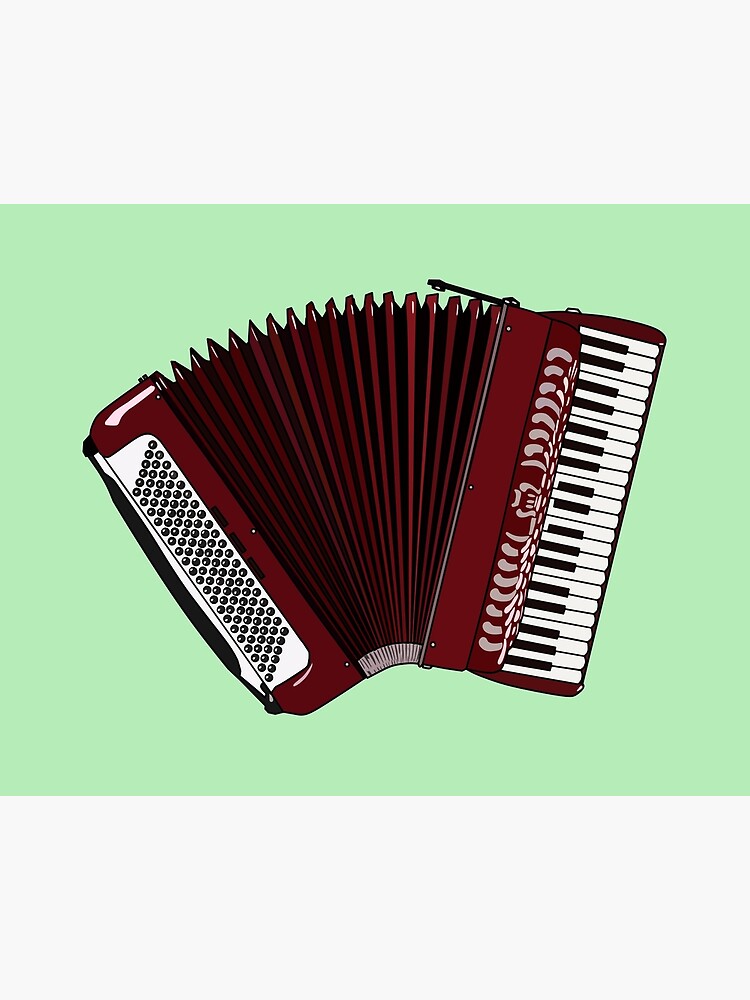This image showcases a beautifully detailed maroon and white piano accordion, displayed in a partially open position. The right side features a classic black and white keyboard, complete with intricately designed controllers situated above the keys, presumably to manage the lifting mechanics. The main body of the accordion boasts a rich maroon hue, creating a striking contrast with the lighter details. On the left side, a series of buttons are visible, whose function remains unclear but may contribute to the instrument's musical capabilities. Additionally, a prominent black strap is attached on the extreme left, accompanied by a smaller strap on the top, indicating mechanisms that allow the accordion to fold and secure properly. This meticulous arrangement hints at the intricate engineering and craftsmanship behind this elegant musical instrument.